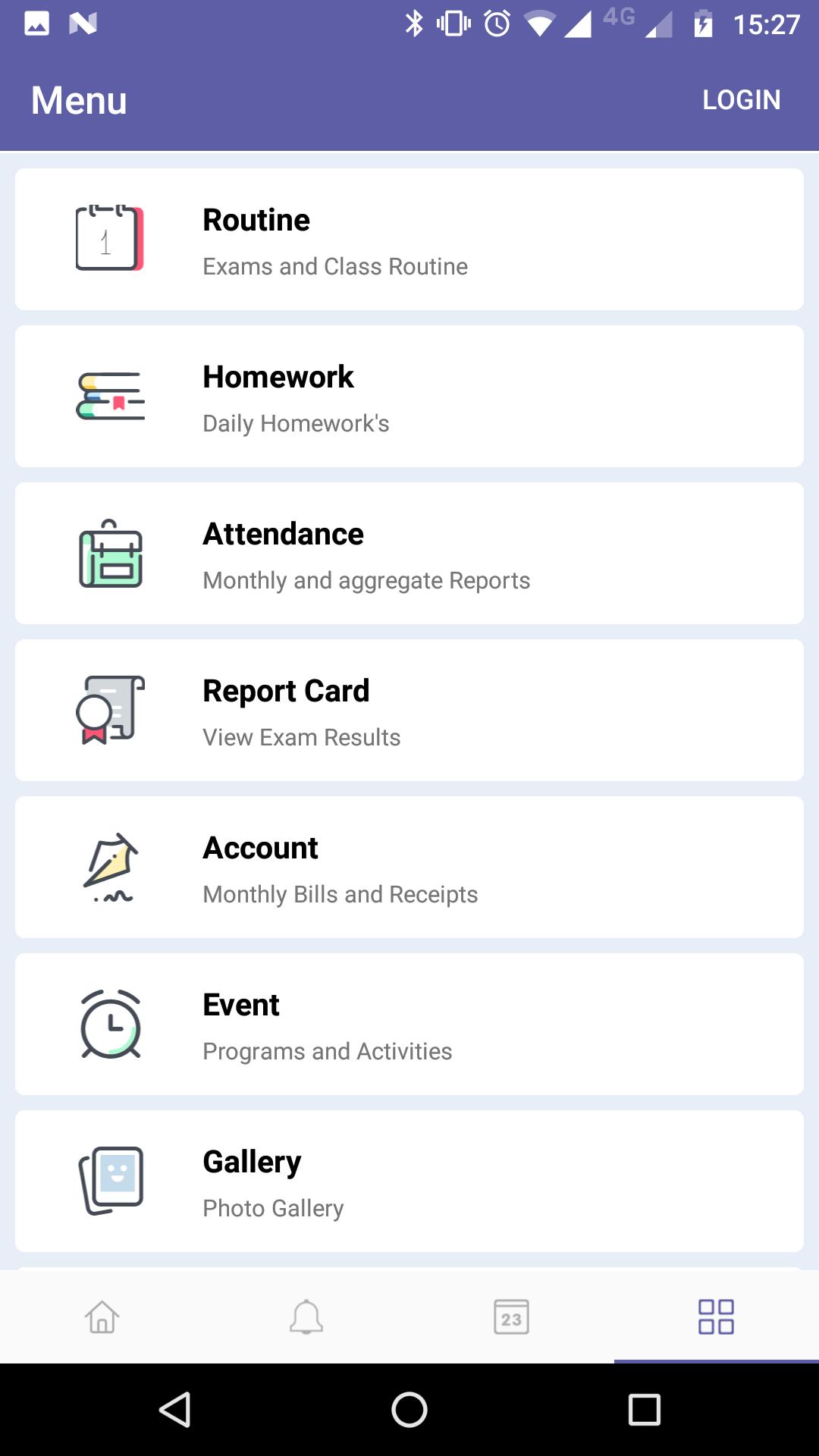The image is a vertically oriented screenshot typical of a smartphone display, featuring a user interface with a predominantly light blue background. The top section of the screen has a distinct purplish hue and contains several white icons. In the upper right corner, icons for Bluetooth, an alarm clock, 4G signal strength, battery life, and the time displayed in military format (15:27) can be observed. 

On the upper left, the text "Menu" is displayed in white, while on the opposite side, "Login" is visible, also in white. Below these, a series of long, white rectangular boxes with icons on their left edges are arranged sequentially. Each box is set against the light blue background and contains bold and less bold text descriptions. They include:

1. **Routine**: exams and class routine
2. **Homework**: daily homework assignments
3. **Attendance**: monthly and aggregate reports
4. **Report Card**: view exam results
5. **Account**: monthly bills and receipts
6. **Event**: programs and activities
7. **Gallery**: photo gallery

At the bottom of the screen, there are navigation buttons: a home button, a bell symbol, a calendar icon, and a grid composed of four small boxes. The very bottom features a black strip with interactive buttons: a triangle pointing left, a circle in the center, and a square on the right.